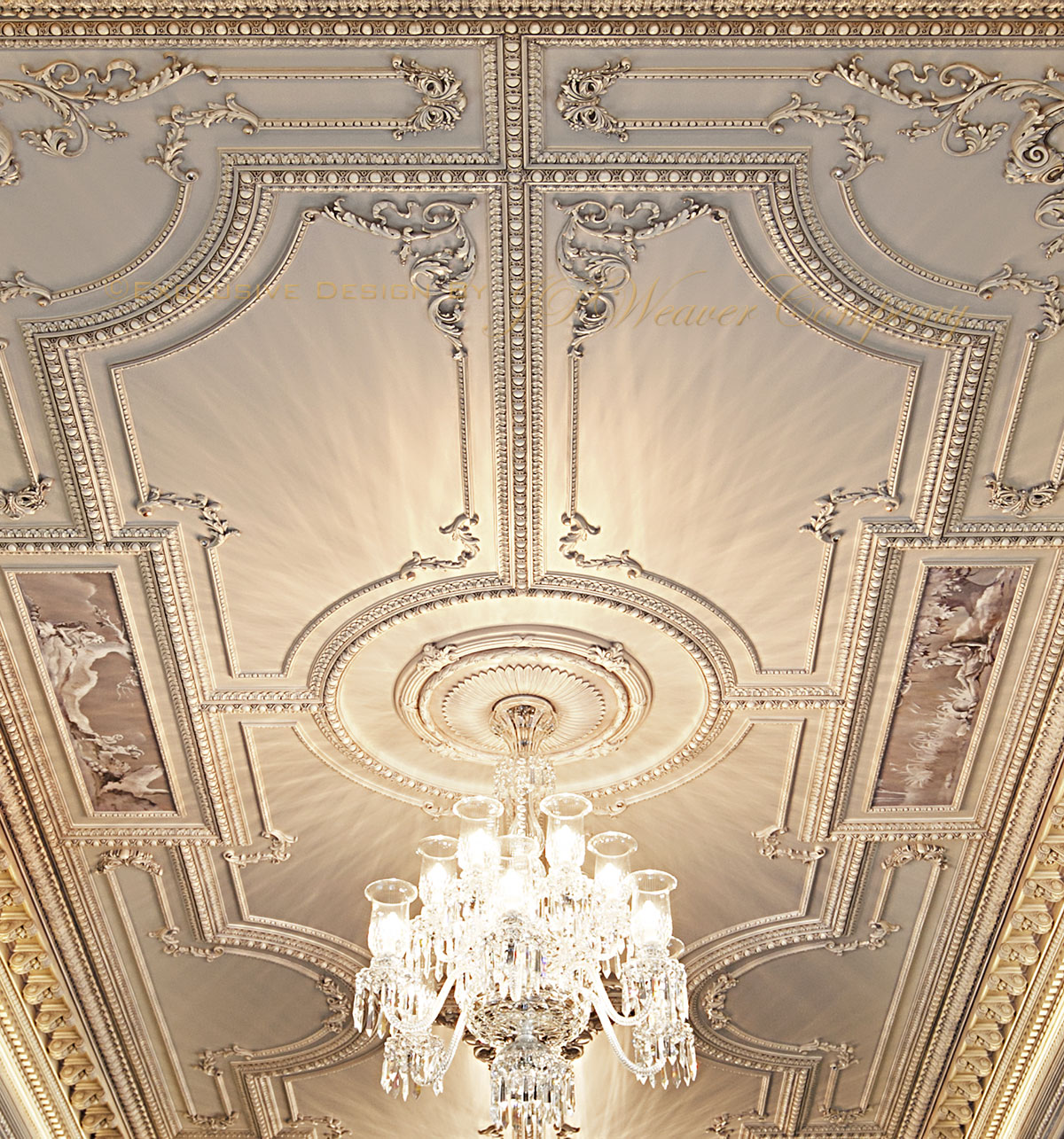This image captures the ornate ceiling of a grand and fancy building, reminiscent of a palace. The ceiling, characterized by an expansive and white surface, features an array of intricate decorative elements, making it appear highly ornate and classy. Central to the design are concentric circular patterns filled with diverse designs and outlines, with some extending outward into semi-circular shapes. Surrounding the border is a well-defined trim with swooshing rectangles and small circles that add to the complexity.

Suspended from the center of these circular patterns is a striking crystal chandelier. The chandelier is not just a functional light fixture but a centerpiece of beauty, featuring glass rods that drape elegantly and numerous cups designed to hold the lights, creating a dazzling effect. Additionally, there are filigree corners that enhance the richness of the overall design.

At the top of the ceiling, there is light text that appears to read "Weaver Company," though the text is somewhat faint and difficult to decipher. The overall decorative ceiling, with its strap work style and detailed moldings, contributes to the impression of an intricately adorned and sophisticated interior space.